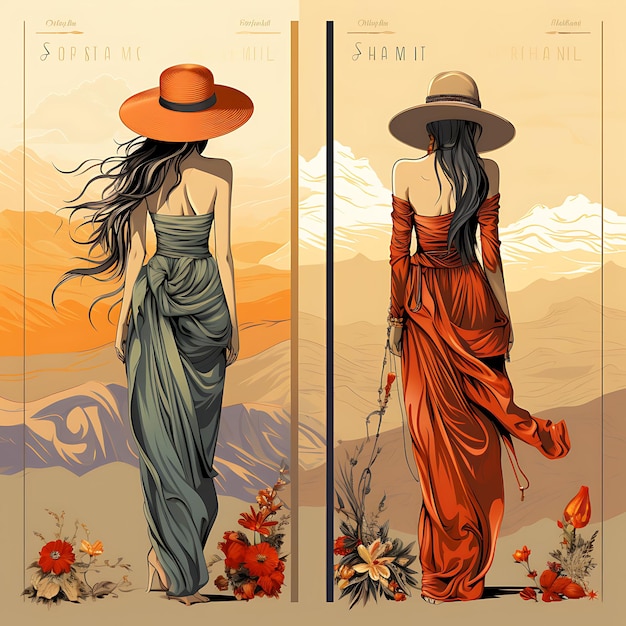This image features a side-by-side display, resembling a collage, possibly found in a magazine or as part of a decorative display. 

On the left side of the display, a woman with long dark hair is depicted from the back, wearing an orange wide-brim hat and a green dress. She is standing in a mountainous landscape, gazing towards the peaks. At her feet, there are red flowers to the right and a red and yellow flower with some greenery to the left.

To the right, a similar scene unfolds with another woman, also viewed from the back and featuring long dark hair. She is adorned with a tan wide-brim hat and a red dress, similarly standing in a mountainous setting. The flowers at her feet include budding red flowers on the right and a yellow flower with greenery to the left.

Both images share a cohesive aesthetic and evoke a sense of serene contemplation amidst nature. At the top of the left image, there is faint text, reading "Shammit" or "Shame it," and the faint text at the top of the right image seems to read "Sophisticate," though this text is somewhat unclear.